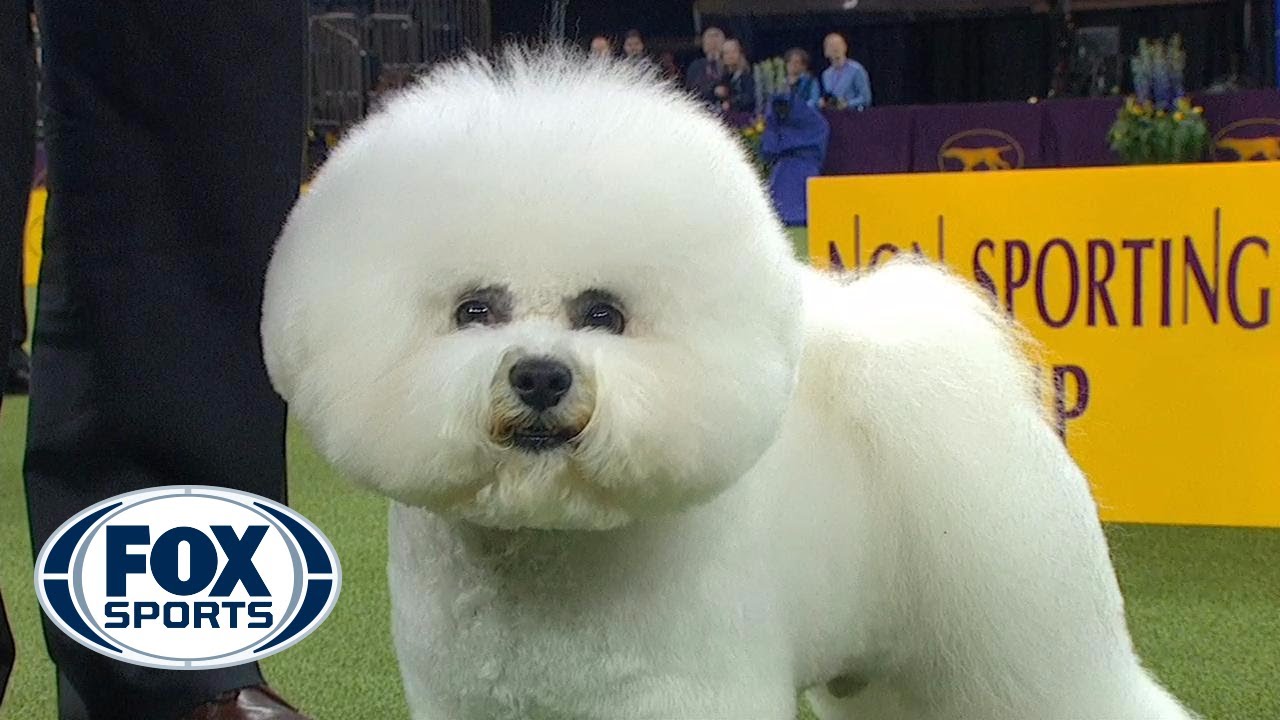This image captures a Bichon Frise at a dog show, prominently positioned in the center of the frame. The dog is remarkably fluffy with an almost perfectly round, cotton-ball-like head, and uniformly trimmed fur that enhances its poofy appearance. Its body is equally fluffy, featuring a floofy tail that arches over its back and spills over the sides. The Bichon Frise has expressive brown eyes, a black nose, and a slight brown stain around its mouth. It looks directly at the camera with an intense gaze. 

In the lower left corner, the blue and white Fox Sports logo is visible, indicating the broadcast source. The dog stands on a green AstroTurf-like surface, suggesting an indoor setting. To the left of the dog, there is a partial view of its handler's leg, clad in navy pants and brown dress shoes. In the background, a yellow sign with purple lettering is partially obscured by the dog, but the legible portion reads “non-sporting group.” Additional details include a purple banner with a yellow dog logo marking the boundary of the ring, and a few people in the background observing the scene, likely judges or spectators.